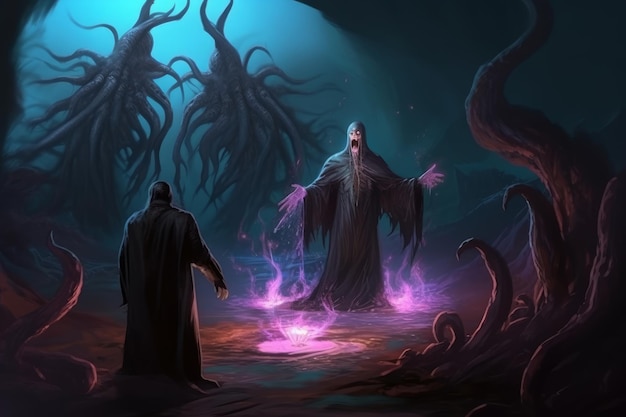This eerie and enigmatic digital artwork depicts a chilling scene reminiscent of dark sorcery or witchcraft. Dominating the center of the image is a sinister figure clad in a long, black robe with flowing, bell-shaped sleeves. His face is ghastly, featuring an open mouth in a terrifying grimace, almost skull-like, exuding an aura of malevolent power. The figure stands amidst a surreal, glowing environment with dark blue, orange, and purple hues, surrounded by three bright, white and purple flames.

In the background, tendril-like shapes, resembling twisted roots or tentacles, stretch ominously, partially illuminated by a turquoise backlight. The scene is further heightened with the presence of an array of strange, intricate plants and possibly alien or animal lifeforms that seem to observe the central figure's ritual.

Facing this menacing sorcerer is another figure, viewed from behind, dressed similarly in a dark garment, his exact features obscured but presenting a shorter, stockier build. Between these two figures floats a radiant, pink jewel, sparking with intense, magical energy, serving as the focal point of the scene. This haunting depiction, steeped in shadows and otherworldly elements, evokes a sense of dark magic and foreboding.